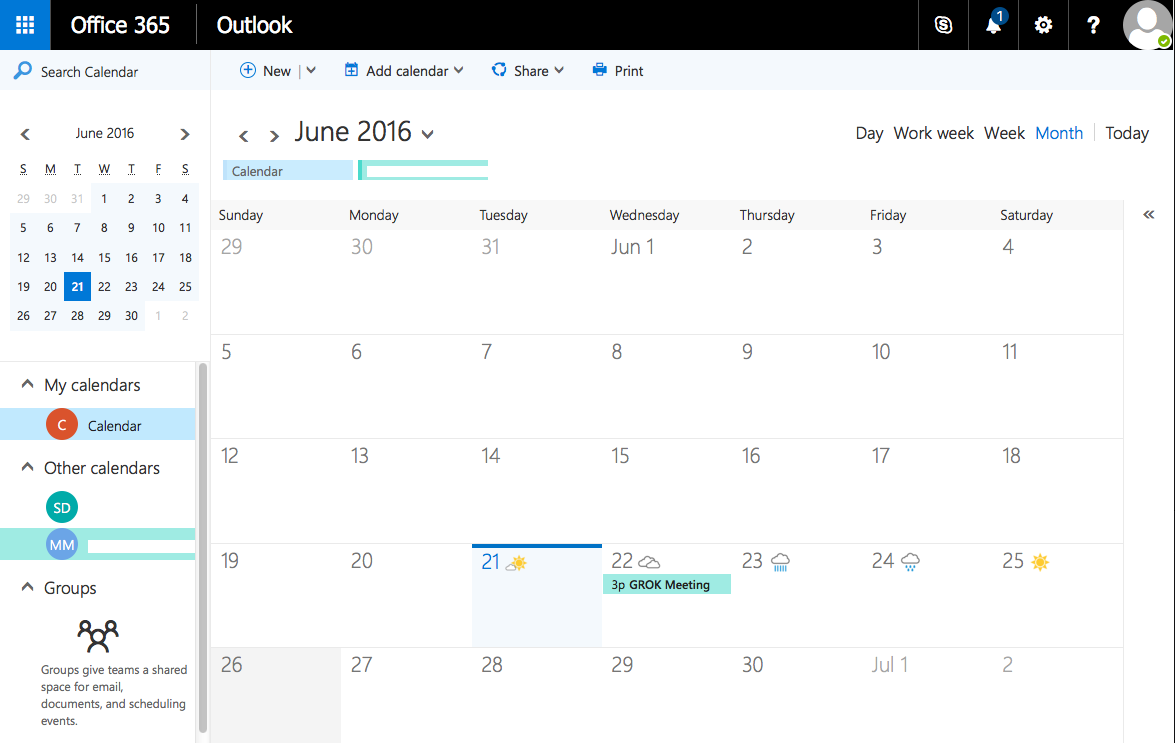This is a screenshot taken from the Office 365 Outlook calendar, specifically focusing on the month of June 2016. The calendar is displaying the dates around June 21st, which marks the first day of summer. There is a scheduled meeting on the calendar for June 22nd, and no other events noted for the remainder of the month. Additionally, the calendar includes weather icons indicating the forecast: rain is expected on the 23rd and 24th, while the 25th is forecasted to be sunny. The depiction of weather is particularly interesting as it adds a layer of practical information for planning and preparation.